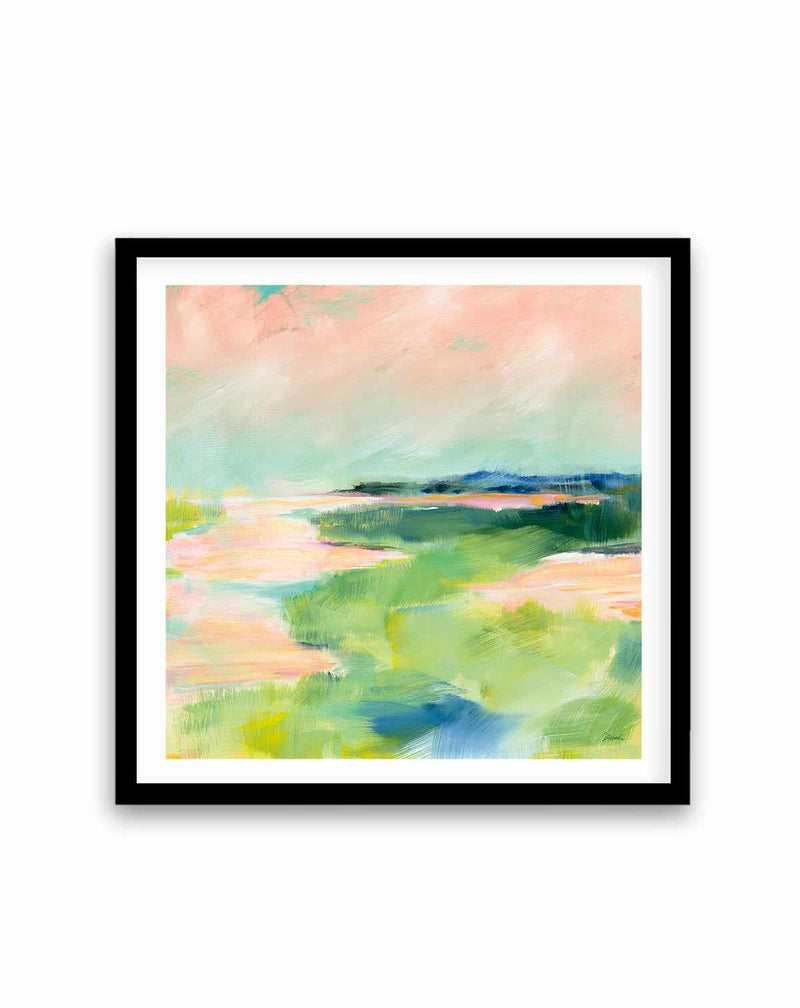This image captures a serene watercolor painting of an outdoor scene, elegantly framed in black and bordered with a white mat. The artwork, with its pastel tones, exudes a dreamy, somewhat abstract feel. The foreground features a blend of greens, yellows, and a touch of blue at the center. On the left, a pink hue suggests either a waterway or a pathway leading toward the horizon, which sits slightly above the middle of the composition. 

The sky transitions from a blue-teal at the bottom to pink clouds above, culminating in a darker teal spot on the top left. On the right side of the horizon, blue hills are visible, fronted by patches of pink and transitioning to darker green, which gradually lightens as it approaches the foreground. The overall aesthetic is a harmonious orchestration of pastel shades, exhibiting the delicacy and fluidity characteristic of watercolor paintings.